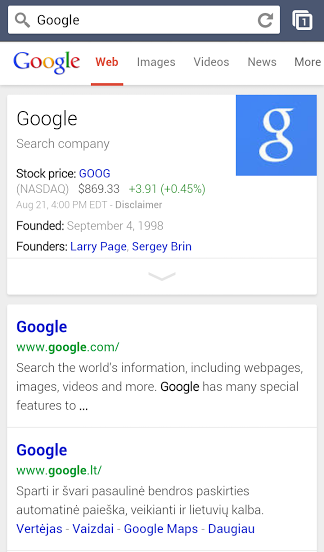A screenshot from a mobile device displays a Google search results page. At the top, a wide search field contains the entry "Google." Below the search field is the Google search banner, accompanied by selectable categories: Web, Images, Videos, News, and More, with "Web" highlighted in red.

The first section under the categories provides information on the company Google, featuring a large blue Google logo, stock values, and a brief history of the company. In the second section, search results for Google are listed, starting with a North American URL for Google, followed by a second option for Google Italy, with the text in Italian.